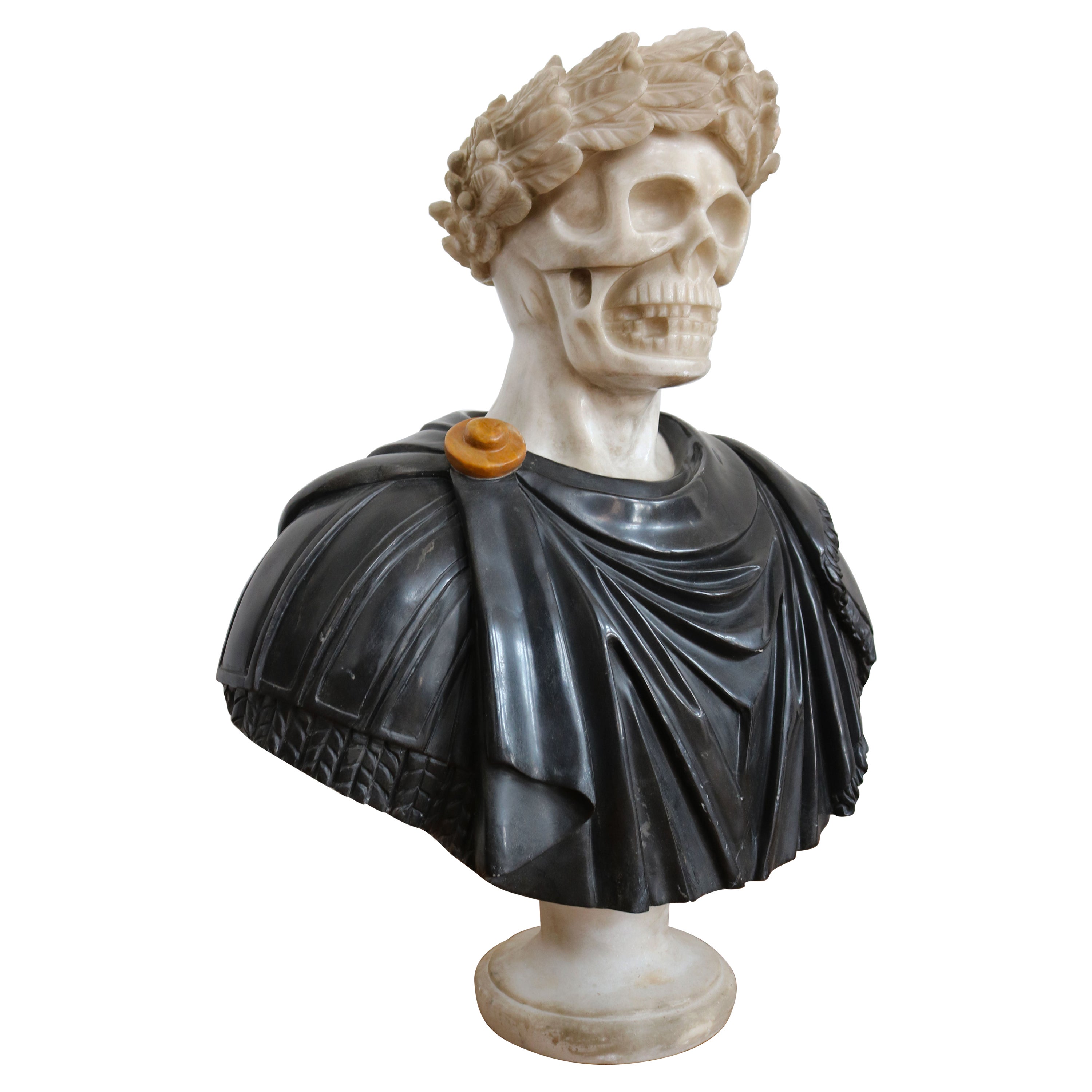This image depicts a detailed bust statue of a skeleton adorned with a blend of classical Greek and Roman elements, crafted to appear like it is carved from marble. The figure, which is positioned against a white background, features a white skull that is missing some teeth and is partially wrapped in a beige-colored headwrap. Atop the skull rests a crown of green leaves, reminiscent of the laurel wreaths worn in ancient Greek times.

Covering the upper torso of the statue, from mid-torso upwards, is intricately sculpted black armor. The armor is designed to mimic a traditional toga, with the fabric gathered at the right shoulder and secured with a brown clasp. Below this clasp, additional black material that resembles chainmail or possibly tire rubber texture can be seen, adding to its detailed and somewhat mysterious appeal. The statue is securely affixed to a stand.

The overall presentation, with its blend of classical and eerie elements, suggests it could serve as a decorative piece, potentially appealing for festive events or as a unique home décor item. Its detailed design hints at it being showcased on an online product page to attract potential buyers seeking thematic decorations.